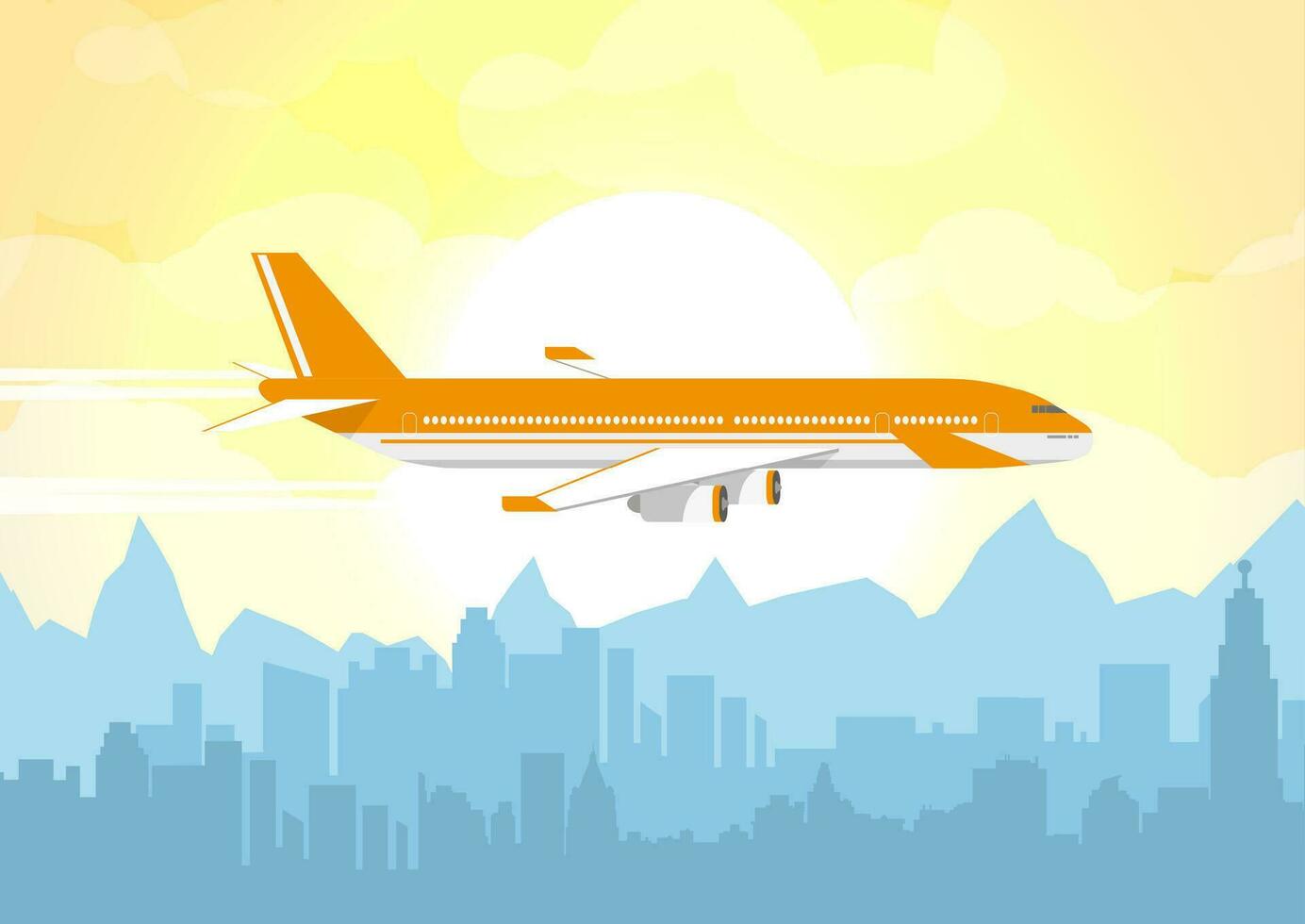The CGI or cartoon image showcases a large passenger plane, characterized by its striking orange and yellow top and blue bottom with white wings and trim, either taking off or preparing to land over a bustling cityscape. The plane glides towards the right side, with a trail of air swirling behind it. The backdrop features a dramatic sun, caught in the moment of either rising or setting, casting a golden hue across the sky. Below, the landscape transitions from the silhouette of mountains in the distance to a sprawling city in the foreground, marked by a mix of skyscrapers and smaller buildings. Scattered clouds add a touch of softness to the vivid sky.